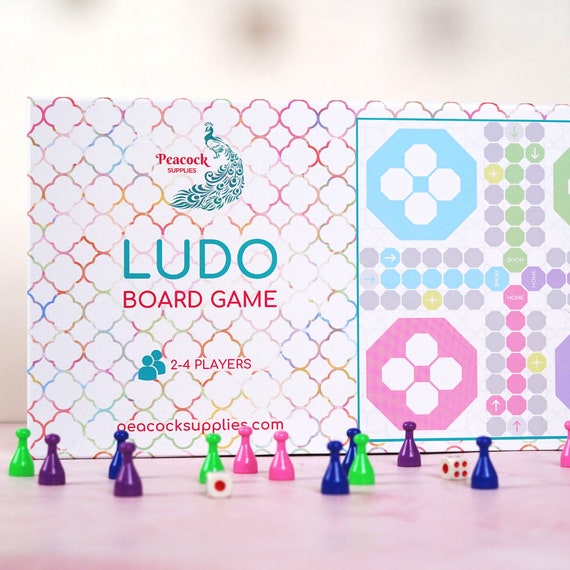This photograph showcases the "Ludo Board Game" by Peacock Supplies, prominently featured with its box standing upright indoors. The top of the box bears the company's name, "Peacock Supplies," along with a teal-colored peacock logo. The game is designed for 2 to 4 players, indicated by two human icons and the text "2-4 players" on the box. The game's board is white, adorned with a colorful geometric pattern in pastel shades of light blue, light pink, purple, light green, yellow, and gray. The word "Ludo" is distinctly written in a bluish-green color. 

In front of the board, on a light pink surface, are various plastic playing pieces in blue, purple, green, and pink, shaped like small cones with bulbous tops resembling miniature bowling pins. Two six-sided dice with red dots are placed among the pieces, displaying combinations of numbers, such as one and four. The background behind the box is blurred and white, drawing focus to the vibrant game components and the meticulous design of the board associated with traditional Ludo gameplay.